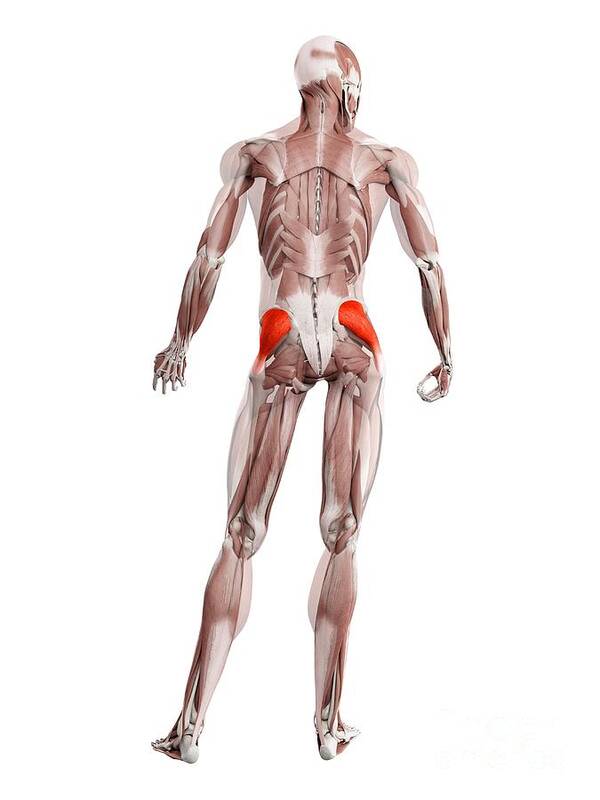The image is a detailed computer-generated diagram of the muscular and skeletal structures of a male human viewed from behind. At the top, the back of the head is visible with a hint of white coloring. As you move downward, you can clearly see the spine in white. Both arms are transparent, revealing the bones within. The diagram meticulously highlights all the bones in the fingers and hands. His hips are prominently highlighted in a bright red color, contrasting with the overall light reddish-brown muscles that cover the body. The leg muscles, including the tendons and gluteal muscles, are also visible with detailed bone structures seen in the thighs, knees, femurs, feet, and toes. The buttocks, or gluteus maximus, are distinctly shown, with two muscles from the hip to the sides of the butt also marked in orange. The diagram provides a thorough representation of muscle groups wrapping around parts of the skeleton, with some white shading indicating exposed bone segments.